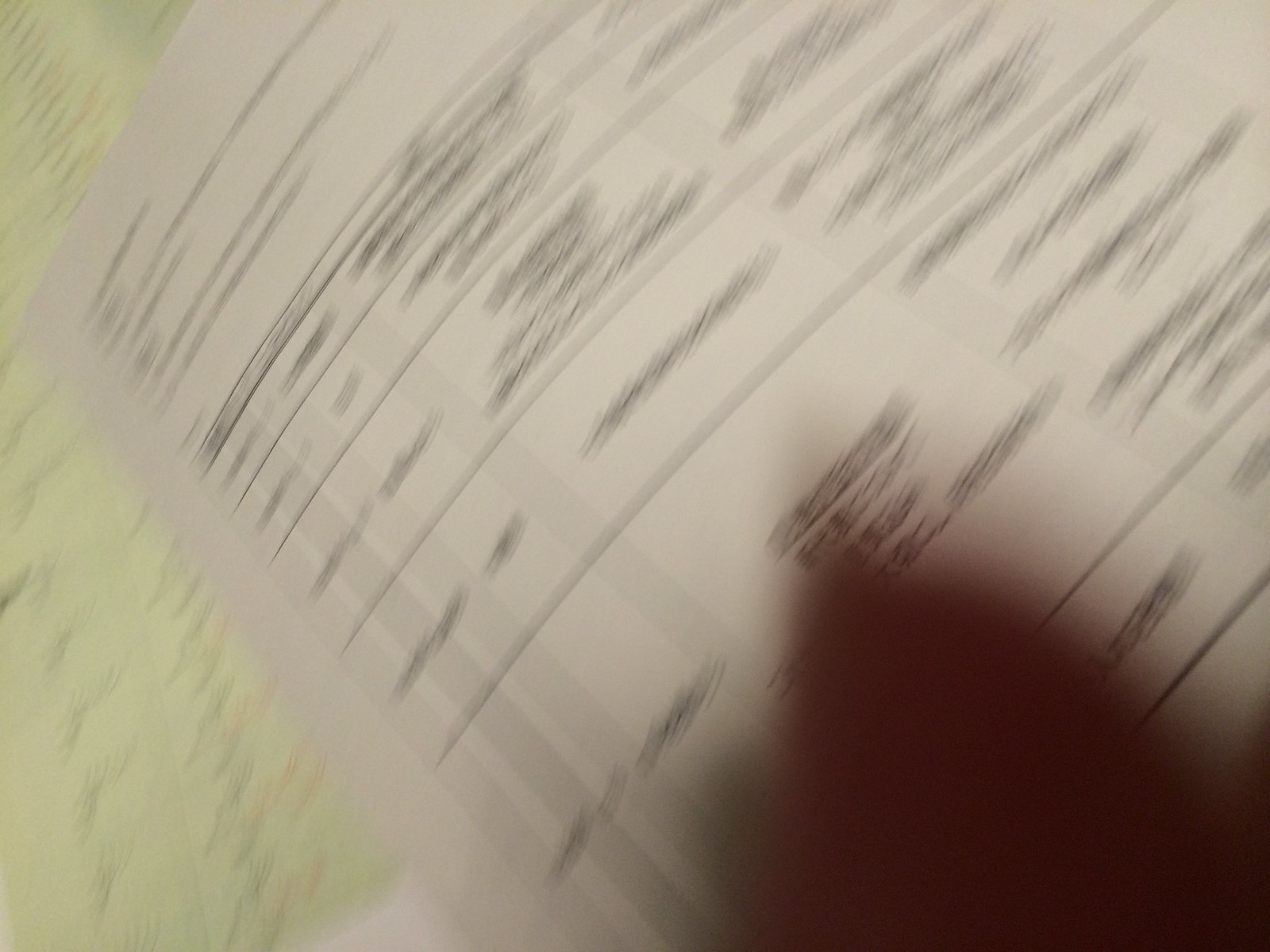This image features a white sheet of paper with multiple lines and columns reminiscent of a structured document, possibly a bill or formal list. The document is extensively redacted, with extensive black scratch marks obscuring all visible text. Positioned diagonally within the frame, the white paper partially overlays a sheet of yellow paper beneath it, which is also filled with illegible scribbles. In the bottom right corner, a blurry, dark shadow resembling a hand hovers over the papers, suggesting someone about to write. The overall scene is one of obscured information and secrecy, with no discernible text due to the extensive redactions.